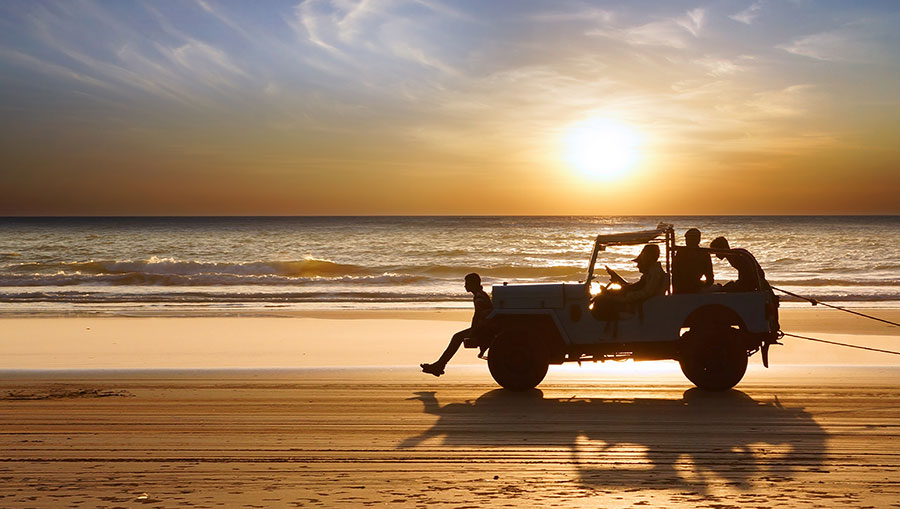On a serene, white sandy beach, an old-school white Jeep is parked near the water's edge under a golden sunset. The sky, painted with muted yellows, oranges, and soft beige hues, contrasts against the light blue backdrop with wispy, elongated clouds adding texture. The ocean waves roll gently onto the shore, their whitecaps illuminated by the setting sun, creating a picturesque scene.

In the front of the Jeep, a person is perched on the lower front fender, while inside, a driver and a passenger are silhouetted against the brilliant backdrop, their identities obscured by the sunlight. The rear of the Jeep hosts two more individuals, likely men, one bent forward, examining something, and the other gazing out toward the horizon. 

A string or rope extends from the back of the Jeep, hinting at the possibility of it towing or pulling something, though the object isn't visible. The Jeep's shadow stretches along the sand, echoing the vehicle's shape and adding depth to the tranquil yet lively image.